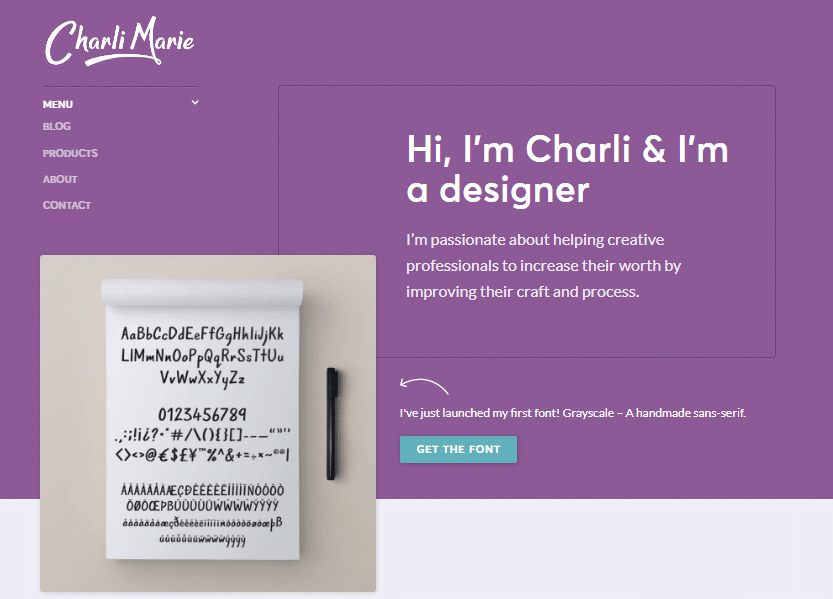The homepage of the website features a purple background with a light gray inset box bordered in white at the bottom. In the upper left-hand corner, the logo "Charlie Marie" is prominently displayed, with a drop-down menu beneath it listing Blog, Products, About, and Contact in white text. The center-right section includes a large introduction: "Hi, I'm Charlie and I'm a designer. I'm passionate about helping creative professionals to increase their worth by improving their craft and process. I've just launched my first font, Grayscale, a handmade sans serif." Adjacent to this text, a curved white arrow directs attention to a beige square area in the lower left, which contains a photograph of a white notepad and a black pen. This pad displays the complete set of "Grayscale" font characters—upper and lowercase letters, numbers, and symbols. Below the introduction, there is an aqua button labeled "Get the Font." The website design effectively showcases Charlie's new font and offers an easy navigation menu.